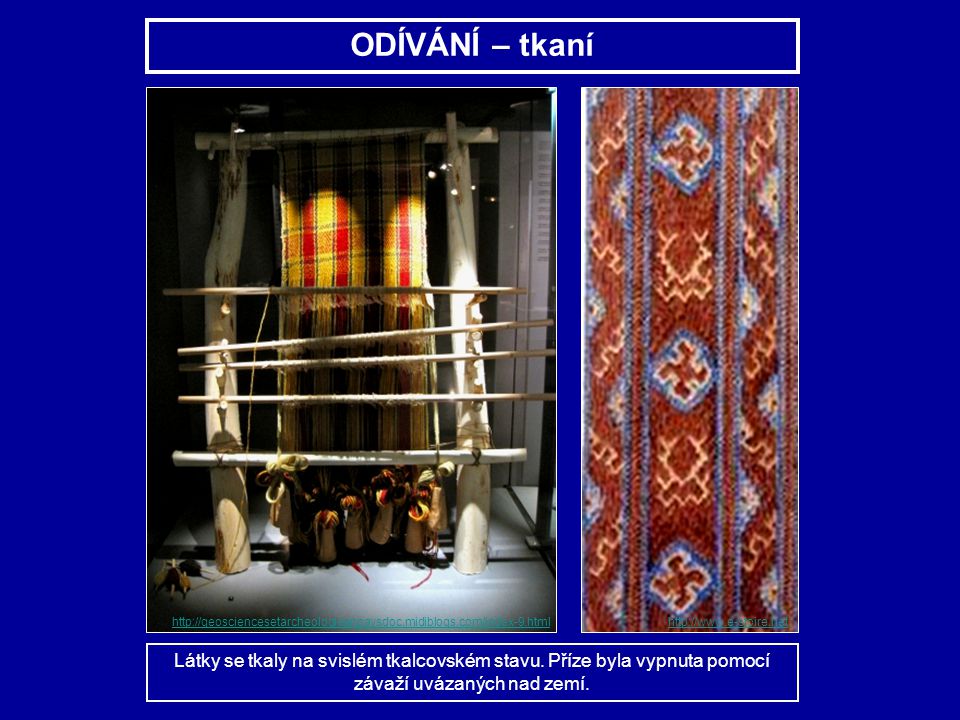The image features a bright blue background with a prominent title framed by a white rectangular outline at the top, reading "ODIVANI-TKANI" in capital letters, followed by lowercase text. This title is in a non-English language. Below this, on the right side, there is a detailed close-up of a reddish-brown fabric with blue and light orange designs, edged in white. On the left side, the image shows an old-fashioned loom with a yellow and red cloth being woven. At the bottom of the image, there is another white-bordered text box containing faint, unreadable text, along with two lines of text in what appears to be Russian. The overall setting hints at a traditional textile or weaving display, possibly showcasing fabrics or rugs with intricate designs and patterns.